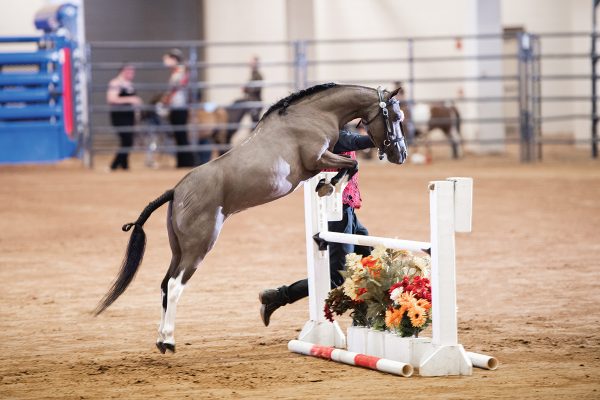In this captivating photograph of an equestrian event, a beautifully groomed, light brown show horse with white legs, a braided black mane, and a tied black tail is captured in mid-leap over a decorated white hurdle. The horse's powerful body arches gracefully, with front legs extended high and rear legs just lifting off the beige dirt ground, exuding strength and elegance. The hurdle, standing about three feet off the ground, features a white rod supported by two vertical beams, with three white-painted cinder blocks adorned with colorful flowers at its base. Behind the leaping horse, a partially obscured handler wearing jeans, brown boots, and a bright red shirt guides the majestic animal. The scene is set within an enclosed equestrian ring, framed by a tall metal fence, where two spectators dressed in black and gray stand to the left, and other horses can be seen in the background, completing the dynamic and picturesque moment.